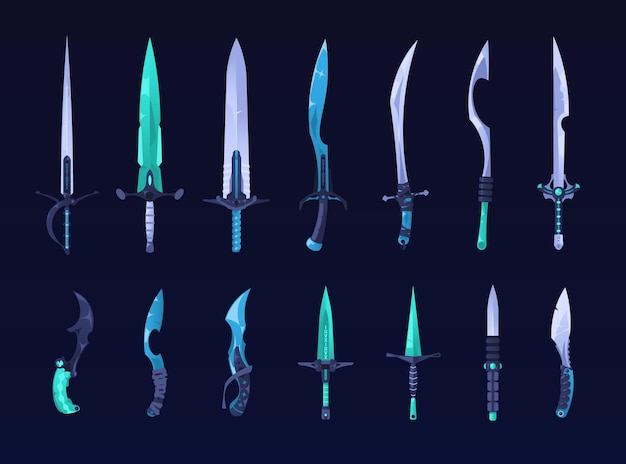The image features a dark, nearly black background, presenting two rows of knives aligned evenly, with seven in the top row and seven in the bottom row, totaling fourteen distinct knives. Each knife exhibits unique attributes; they differ in shape, blade length, handle design, and colors. The blades appear in vibrant hues including purple, green, yellow, pink, and orange, emphasizing their intricate designs and various points, notches, and hook sections. The knives on the top row have longer blades compared to the ones on the bottom row, which feature shorter blades and more varied handles. These details suggest that the collection might belong to a weaponry enthusiast or a collector of fantastical, fantasy-inspired blades, rather than practical everyday pocket knives. Bright lighting accentuates the shining blades against the backdrop, making them appear almost surreal or like artifacts from a fantasy world.